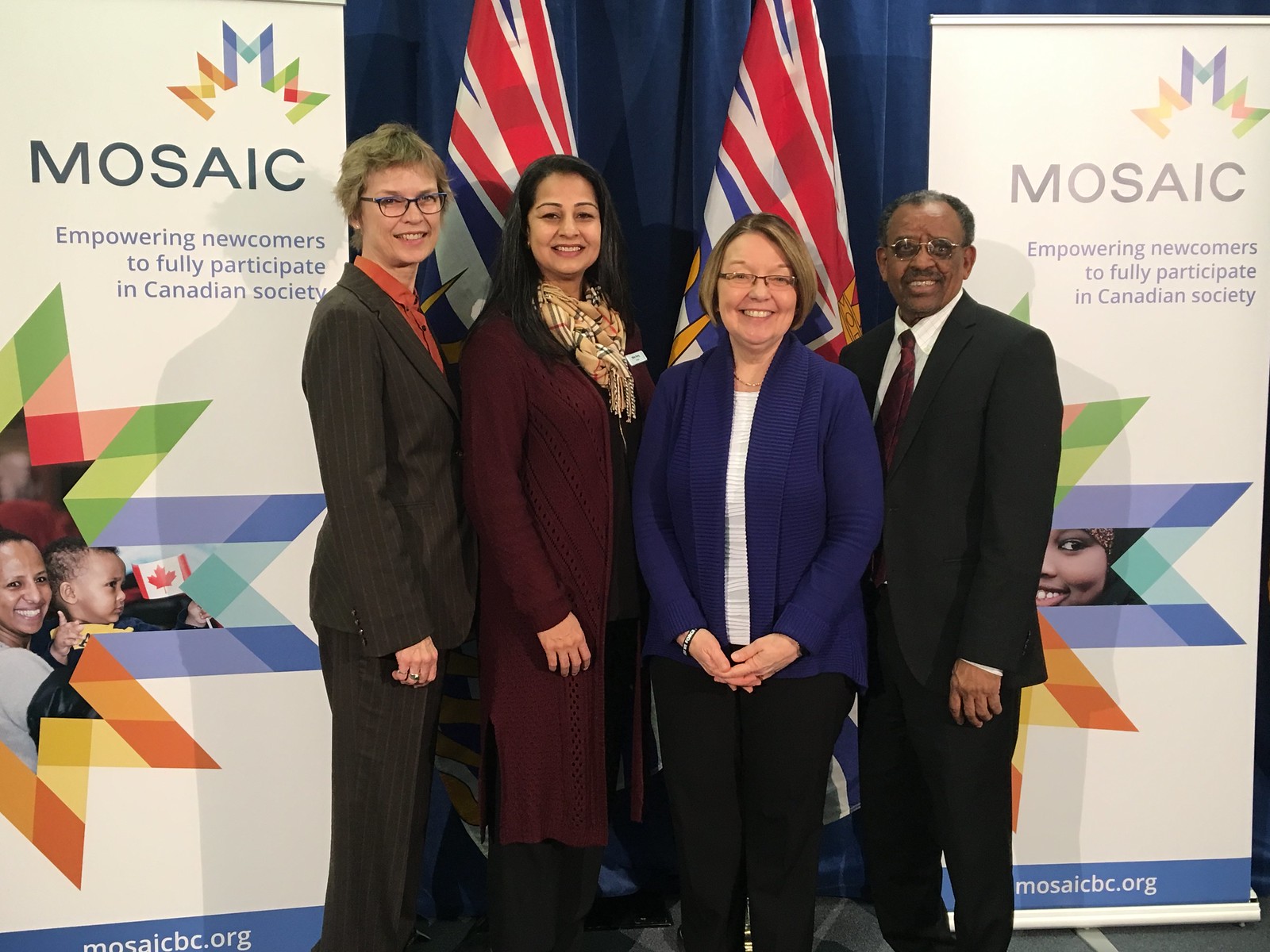In this image, four individuals, three women and one man, are standing together, all dressed formally. They appear to be in their 40s and are likely attending an award ceremony. The woman on the far left is wearing a gray suit with an orange shirt underneath, has short blonde hair, and glasses. Next to her stands a woman of Indian descent, clad in a purple jacket, black pants, and a scarf. The third person is a white woman with short blonde hair, dressed in a blue jacket and black pants. On the far right is a man of Indian descent, wearing a black suit with a burgundy tie and glasses. They are posed in front of two partially obscured flags, with prominent signs on either side that read, "Mosaic, empowering newcomers to fully participate in Canadian society."